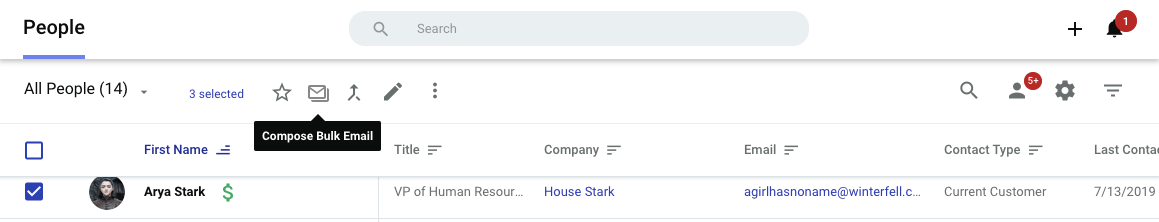The screenshot appears to be from People magazine's website or an associated application interface. The interface layout is straightforward with recognizable elements. The text is printed in small black font. At the center of the top section, there is a search bar. To the right, there is an alert icon represented by a black bell with a red circle displaying the number "1." Directly underneath, the page displays the text "All people" and "14," with "3 selected" highlighted in blue. This section also includes several icons: one for composing bulk emails, a star, and two unfamiliar icons. A menu is present as well.

One of the entries in the list is checked, revealing the details of an individual named Ara Stark. Her profile picture shows her to be a white woman. Her title is "VP of Human Resources" at "House Stark." Additionally, her lengthy email address and her contact classification as a "current customer" are visible, along with the last contact date of July 13, 2019. There's also an indication of alerts and new messages, evident from the person icon and an accompanying notification.